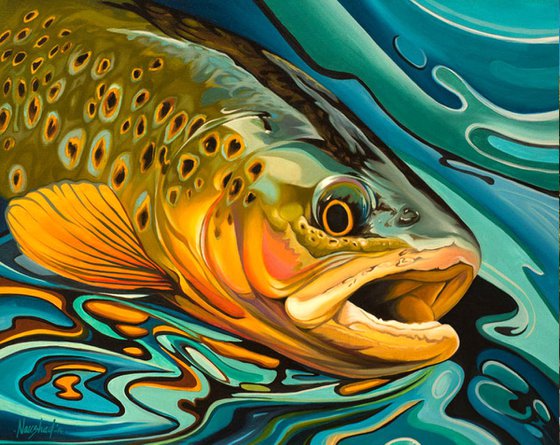The image showcases a somewhat abstract, colored drawing or painting of a fish that appears to be mid-motion. The fish's back extends off the upper left corner of the frame while its mouth, wide open and seemingly struggling for breath, points toward the lower right corner but does not quite reach it. The fish, possibly a trout, displays a reflective surface along its dark-green back and is adorned with distinctive yellow dots with black centers, some encircled by light blue. Its right eye is visible, just right of the center of the image, surrounded by yellow and black. One fin can be seen on the left side of the fish's body within the composition. 

The background of the artwork suggests an abstract portrayal of water, with an oily texture created by swooshing strokes. The water features a diverse palette with shades of blue, green, turquoise, and black swooshes interspersed with occasional orange. The upper parts are more dominated by these cool tones in curves and stripes. Overall, the backdrop creates a dynamic and swirling visual effect, enhancing the impression of the fish's motion within its aquatic environment.